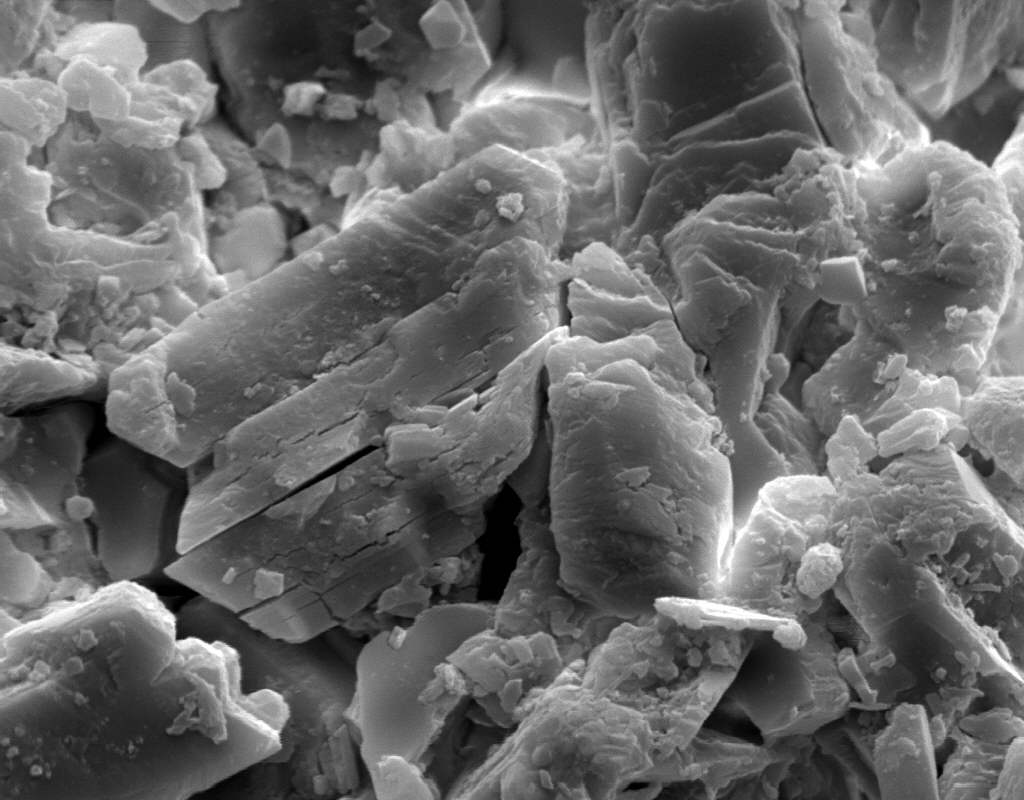This black and white microscopic photograph captures an intricate, highly magnified flaky surface with remarkable detail. The image reveals a complex landscape of overlapping layers, akin to a mosaic of brittle shards and fragments. High contrast lighting accentuates the irregular, yet predominantly straight-edged pieces, emphasizing severe textures and fissures across the surface. The photograph evokes the appearance of various possible materials such as minerals, rocks, shell fragments, or perhaps even skin cells, all under extreme magnification. The illuminated edges suggest a light source from above, highlighting the layers and segments in stark relief against the grayscale backdrop. Despite the uncertainty about the exact nature of the subject, the photograph vividly showcases a fragmented, flaking surface with both broken and intact elements, giving a surreal glimpse into a miniature, layered world.